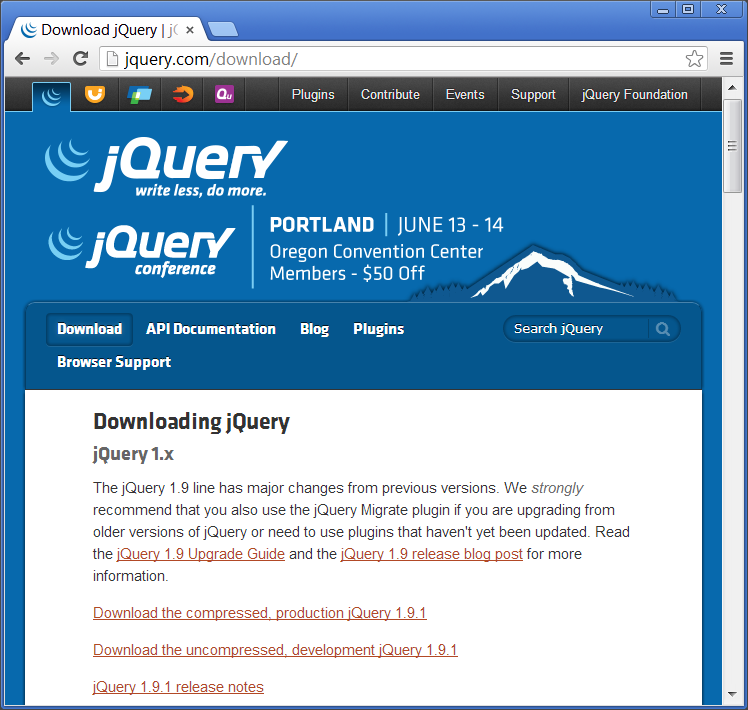This is an image depicting a slightly outdated website focused on the jQuery library. The website's layout is primarily square with a predominant blue and white color scheme. At the top of the image is a grey address bar containing the URL in black font: jquery.com/download/. Inside the address bar is a white search bar with a file icon beside it.

The central portion of the image features a blue background prominently displaying the jQuery logo - a series of blue, half-moon shapes that decrease in size from bottom to top. Next to the logo, "jquery" is written in lowercase, followed by the slogan "write less, do more."

Directly beneath this, there is a section titled "jQuery Conference" with details outlined within a bordered area. It mentions an event taking place in Portland, Oregon, on June 13 and 14 at the Oregon Convention Center, with a special discount of $50 for members. This section is separated by a thin vertical blue line.

Below the event information is a white download box. It mentions "Downloading jQuery 1.x" with a note about significant changes in version 1.9 compared to previous versions. Users are strongly encouraged to use the jQuery Migrate Plugin if upgrading from older versions or if they need to use plugins that haven't been updated. The box lists various terms and reasons for downloading the jQuery library, which appears to be intended for web development and plugin compatibility.

Overall, the image gives a detailed look at a download page for the jQuery library, complete with event information and download guidance.